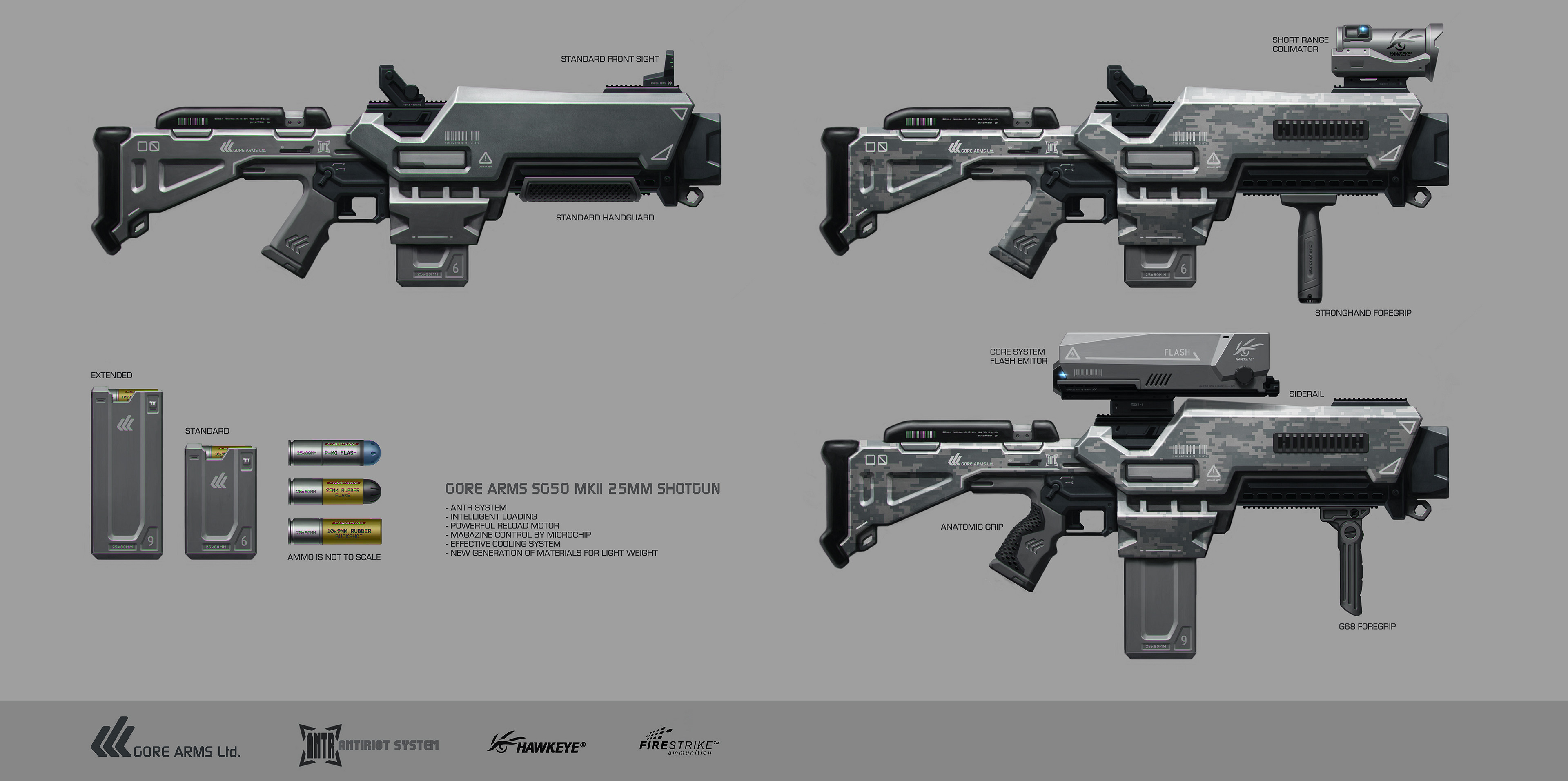The image is a detailed color illustration in landscape orientation, showcasing three futuristic, sci-fi-esque shotguns with various attachments and ammunition. Positioned in the top left, the first gun features a standard front sight and handrail, maintaining a classic appearance with a digital twist. Next to it on the right, the second gun stands out with its digital camo paint, labeled as having a Short Range Culminator and a Strong Hand Foregrip, which is visibly attached to the gun. On the bottom right is a more advanced variant, equipped with a Core System Flash Emanator scope, Side Rail, Anatomic Grip, and a G68 Foregrip. The caption below this gun reads "Gore Arms SG50MK2 25mm Shotgun," emphasizing its sophisticated design. The bottom left corner highlights various ammunition types, including two bullet casings and three individual bullets, providing a comprehensive view of the weapon’s capabilities. The image's background features a dark gray horizontal band with black logos, enhancing the overall futuristic and graphic design aesthetic.